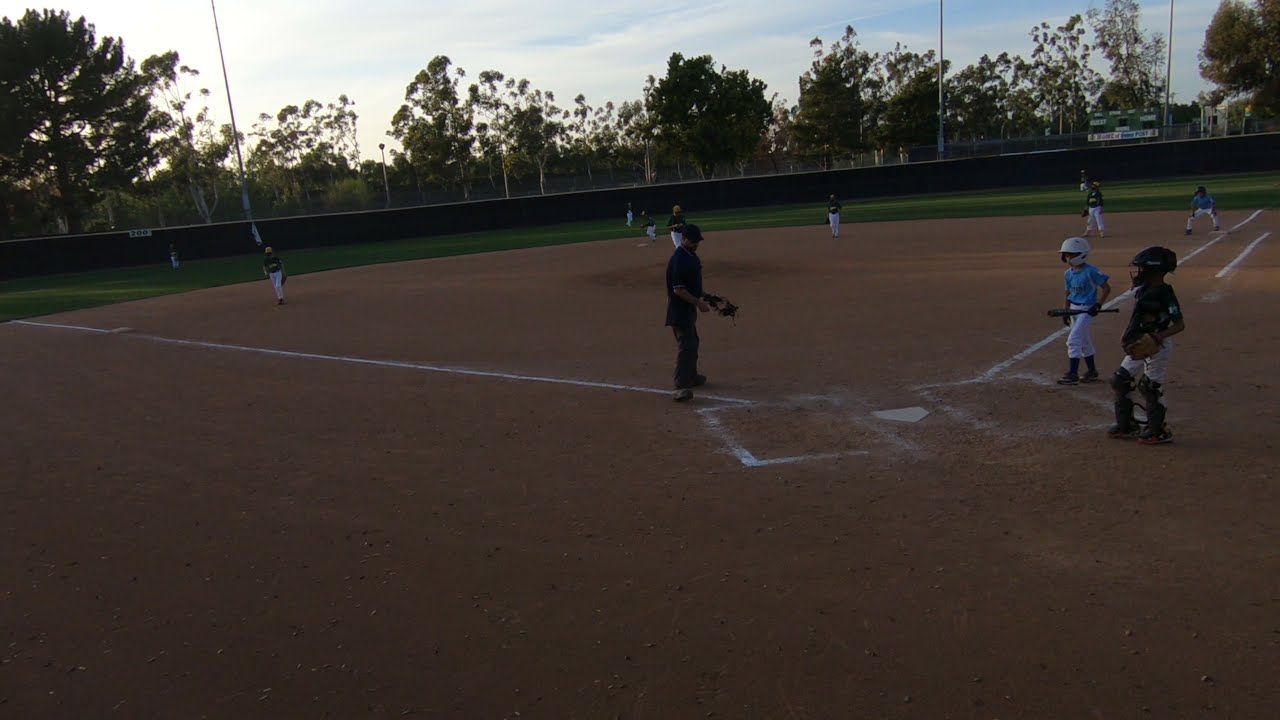This is an outdoor photograph capturing a little league baseball game taken from just to the left behind home plate, likely near sunset as the lighting is low. The sandy-colored baseball diamond has white lines extending from home plate to each base. In the scene, there's an adult umpire positioned just outside the left-hand batter's box, watching over the play. A young batter, dressed in a blue shirt, white pants, and a white helmet, is walking into the right-hand batter's box, while the catcher, outfitted in white pants and all-black gear, stands ready and looks towards the umpire. In the background, the outfield features green grass and a short dark wall, with trees and a scoreboard visible beyond it. The photo captures the calm pre-game moments, with an overarching ambiance of the late afternoon sun casting a softer, slightly shadowed light over the field.